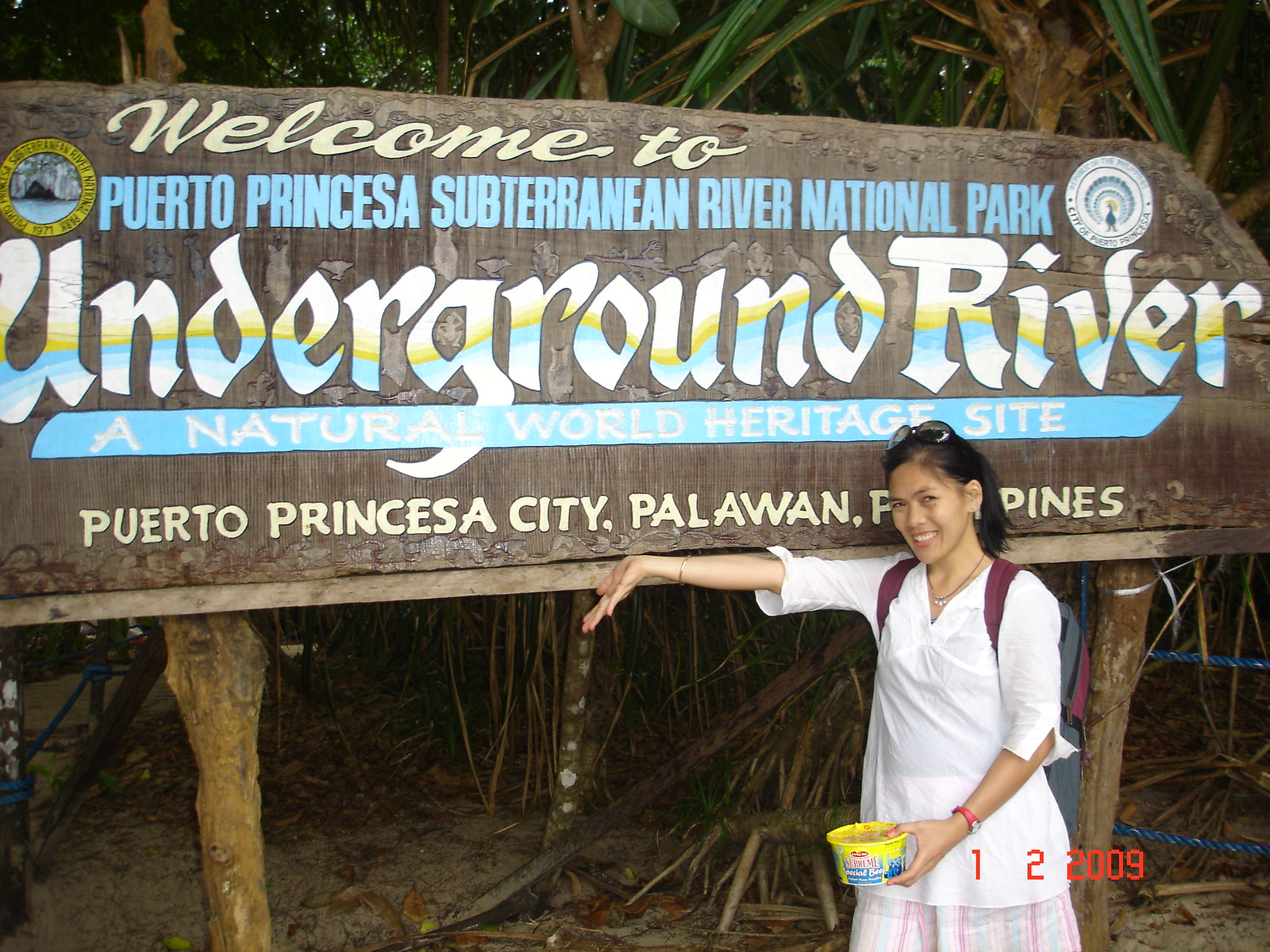The photograph captures a young woman standing in front of a large wooden sign, reading "Welcome to Puerto Princesa Subterranean River National Park, Underground River Natural World Heritage Site, Puerto Princesa City, Palawan, Philippines." The text on the sign is interrupted by her head, but most details are clear. She is smiling at the camera, her dark hair pulled back with sunglasses perched on top. She wears a white shirt and a maroon and brown backpack, with light-colored pants or a skirt. 

In her left hand, she is holding a yellow bowl near her stomach while her right arm is outstretched, pointing towards the sign. The image shows thick tropical vegetation in the background, with mostly brown tree trunks and some green leaves. A wristwatch adorns her left wrist. The date "1-2-2009" is prominently displayed in red at the bottom of the image, indicating it was taken on January 2, 2009.